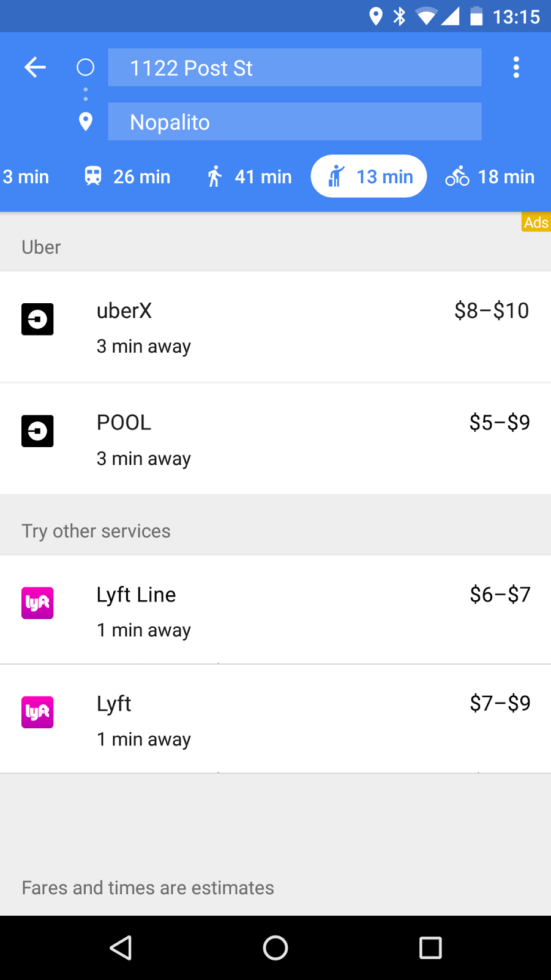This is a detailed screenshot from a cell phone displaying travel options and their estimated times. At the top right corner, icons for location, Bluetooth, Wi-Fi, and battery status are visible. The time is displayed as 13:15. Below this, a blue banner shows directions from "1122 Post Street to Nopalito." The travel options are as follows: 

- Bus: 26 minutes
- Walking: 41 minutes
- Rideshare: 13 minutes
- Bicycling: 18 minutes

For rideshare services, specific options are provided with time and cost estimates:

- Uber: 3 minutes away, priced between $8 to $10
- Uber Pool: 3 minutes away, priced between $5 to $9
- Lyft Line: 1 minute away, priced between $6 to $7
- Lyft: 1 minute away, priced between $7 to $9

All measures and times mentioned are estimates. The image is a vertical screenshot without any photographic elements, people, animals, plants, buildings, or vehicles such as motorcycles, airplanes, or helicopters.